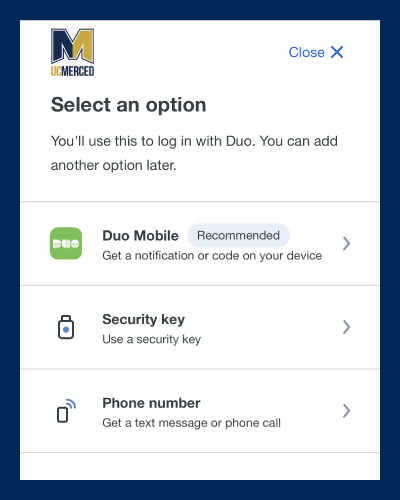The image displays a pop-up login interface, likely intended for a phone or computer screen, featuring a distinctive navy blue border and a white background. 

In the upper left corner, the UC Merced logo is prominently displayed. The logo consists of an "M" that is divided into blue (top half) and gold (bottom half) segments, with the letters "UC" in gold and "Merced" in blue beneath it.

To the left of this logo, there's a blue 'close' button. Below the logo, in a lighter gray font, are the instructions: "Select an option. You'll use this to log in with Duo. You can add another option later."

Three login options are presented beneath the instructions:

1. **Duo Mobile** (recommended), with a Duo logo and a brief explanation stating you can receive a notification on your device. A clickable button allows users to select this option.
   
2. **Security Key**, accompanied by a key icon, and an instruction to "Use security key." This option also features a clickable button.

3. **Phone Number**, illustrated with a phone icon emitting signal bars, offering the options to "Get a text message or phone call." This too includes a clickable button for selection.

The layout and design emphasize the seamless user experience of logging in through Duo with multiple authentication methods.